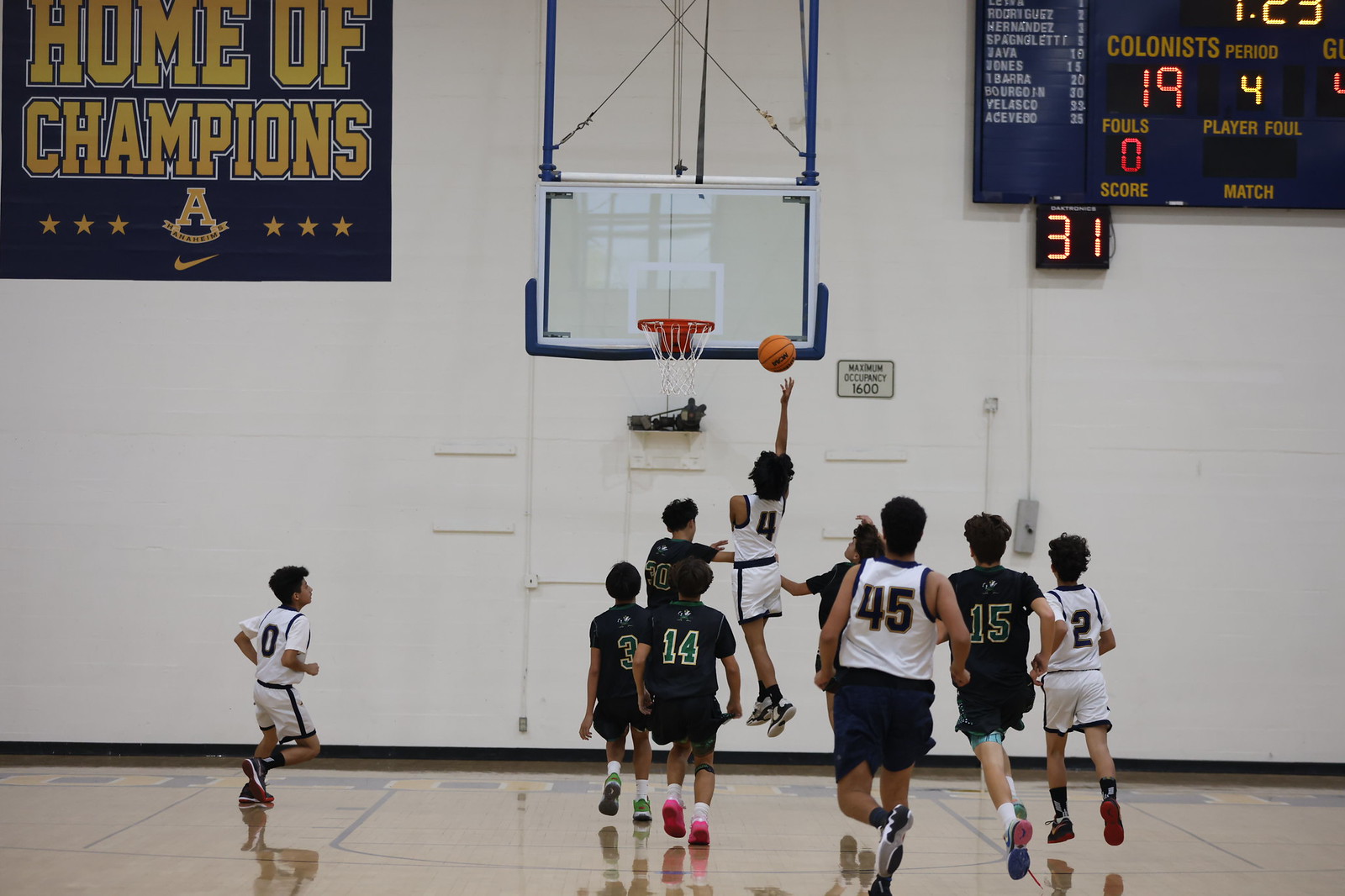The photograph captures an intense moment in a youth basketball game, set on a brownish court with a white wall as the backdrop. At the center of the image, player number 4 from the team in white jerseys is captured mid-air, attempting a layup towards the clear glass backboard and red metal hoop. Surrounding him are players from both teams—approximately four to five boys in white jerseys featuring numbers 45, 15, 14, 2, and 0, and five boys in dark jerseys, possibly black or navy blue. In the upper left corner of the image, a blue and yellow banner reads "Home of Champions," adorned with stars and a large letter 'A.' In the upper right corner, a partially visible scoreboard shows the home team, the Colonists, leading with 19 points in the fourth period, and a shot clock displaying 31 seconds remaining. The dynamic composition and surrounding details vividly convey the excitement and atmosphere of the game.